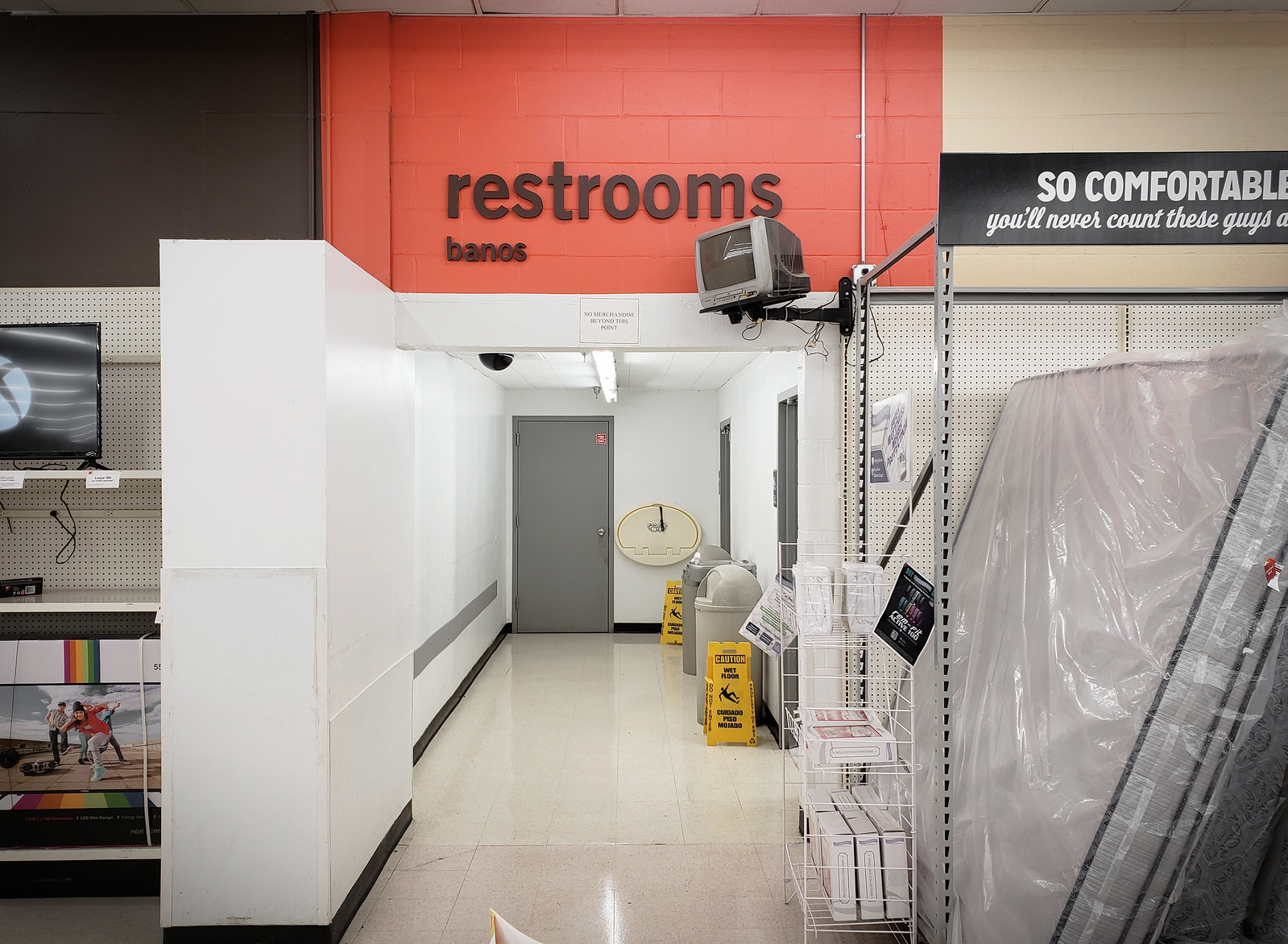This image depicts a hallway in a retail store leading to the restrooms. The store has polished white tile flooring and a drop-tile ceiling, with the left side of the hallway featuring white metal shelves and a section where the ceiling is painted black. The right side of the hallway displays mattresses wrapped in plastic under a sign that reads, "So comfortable you'll never count these guys again," suggesting the presence of a sheep mascot that is not visible in the image. The focal point is the brightly painted orange upper wall in the center, which clearly directs to the restrooms with the text “Restrooms, Banos” displayed prominently. Below this, a hallway painted white extends backward, featuring three heavy gray metal doors, presumably leading to the bathrooms as indicated by placards outside them. There are also two slippery wet floor caution signs and two large gray metal trash cans, similar to those seen in schools, placed in front of the doors. Additionally, a drinking fountain is positioned near the restrooms. Above the restroom doors, an old-style TV, currently turned off, is mounted, possibly for security purposes. The combined details suggest a non-American retail setting, likely from an era when flat-screen televisions were becoming common.